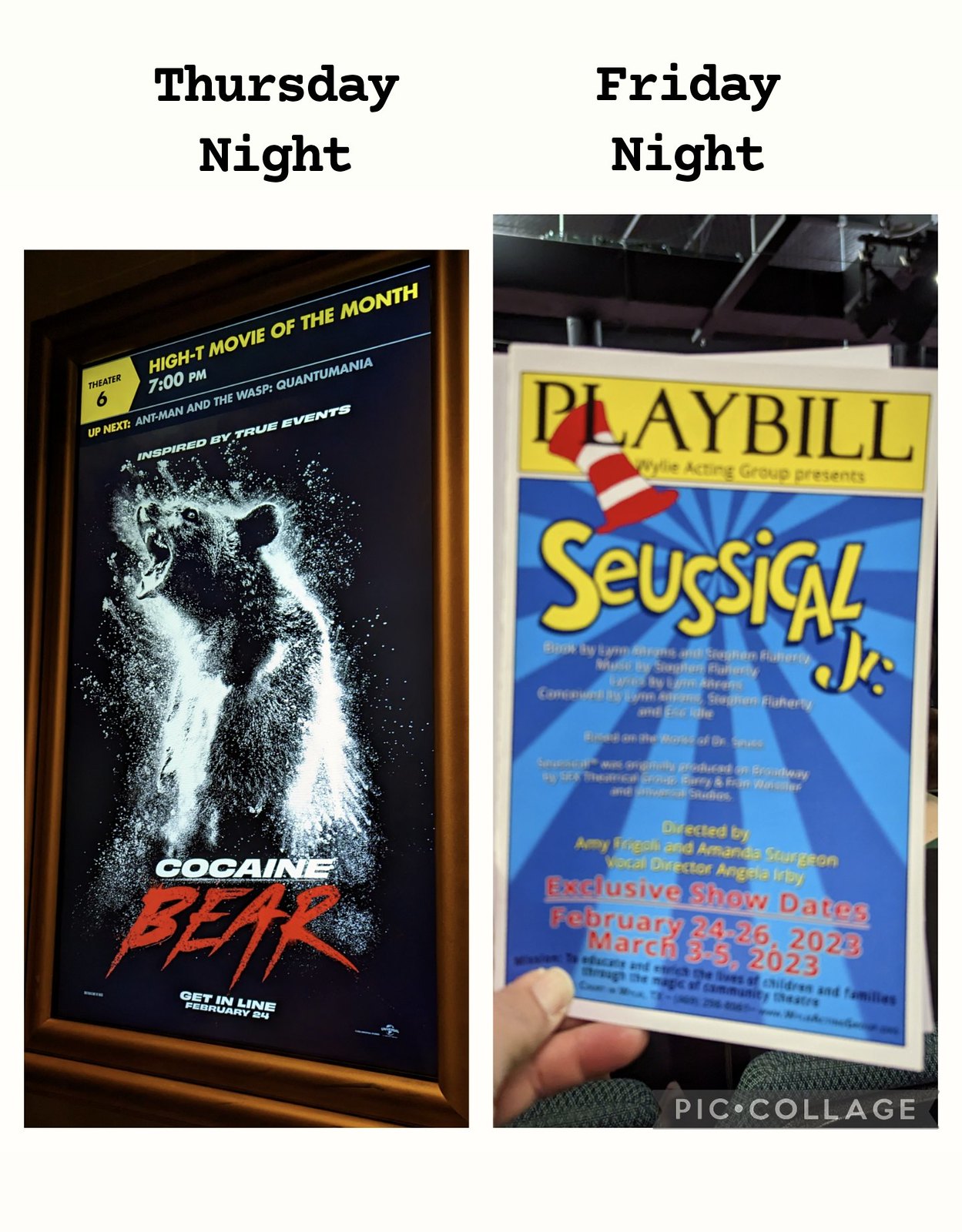This image is a detailed collage showcasing two entertainment events. On the left side, there's a focused area that starts with the text "Thursday Night" at the top left corner. Below it is an advertisement for a movie night featuring the film "Cocaine Bear" at Theater 6, billed as the Hi-Tea Movie of the Month. The poster, which is cast against a black background, prominently displays an image of a roaring bear with the text "Inspired by True Events" above. In bold red and white, it says "Cocaine Bear" with a call to "Get In Line" at Theater 24. The event is scheduled for 7:00 pm; the poster also mentions that "Ant-Man and the Wasp: Quantumania" is coming up next. 

On the right side of the collage, it reads "Friday Night" at the top right corner. Below this, there's an image of a playbill for the stage play "Seussical Jr.," presented by the Wiley Acting Group. The playbill announces exclusive show dates: February 24th through 26th, 2023, and March 3rd through 5th, 2023. The text is primarily yellow and red with additional smaller text in black. Both parts of the collage provide a vibrant glimpse into the diverse entertainment offerings available over two nights.